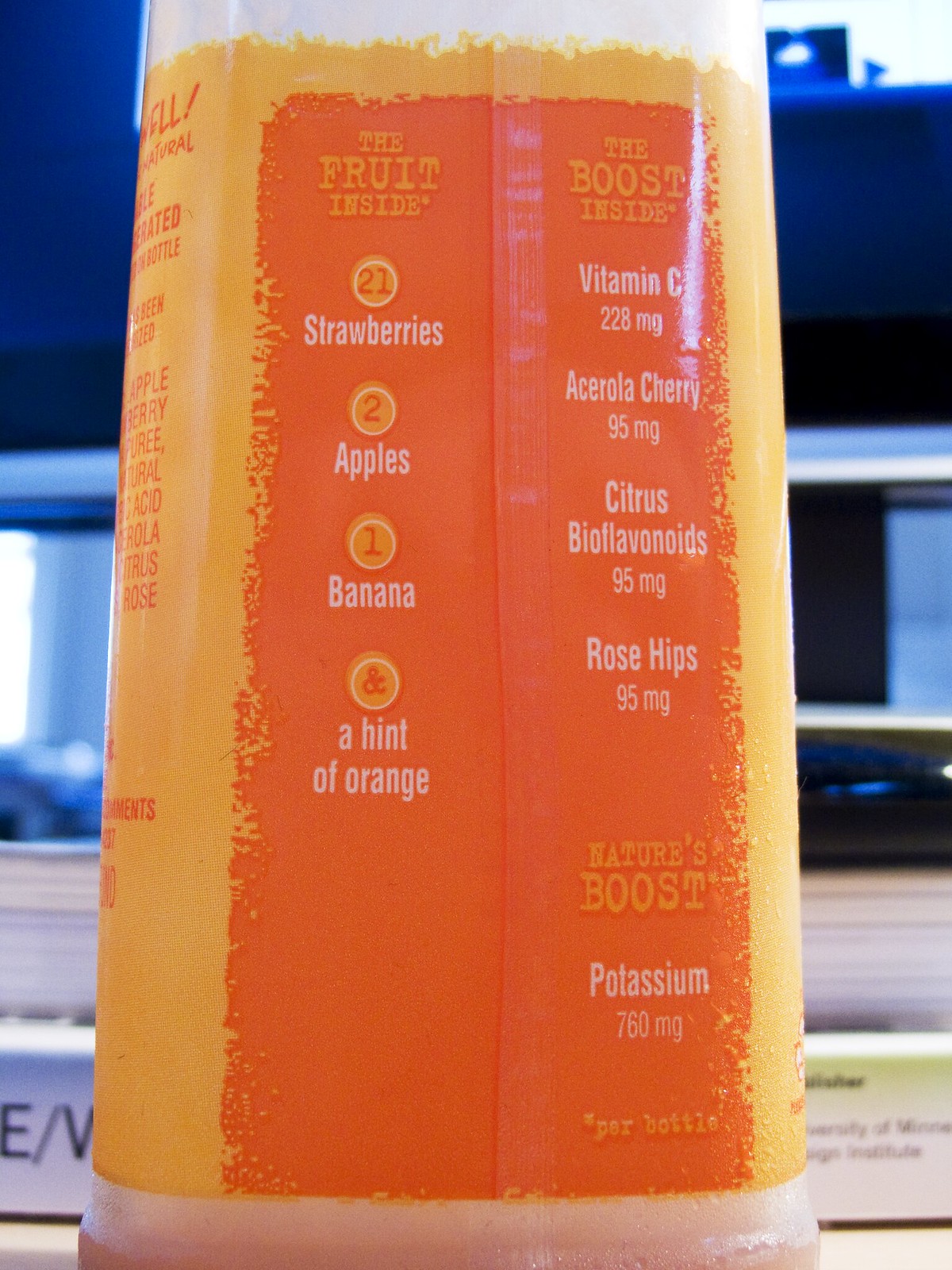This image features a close-up view of the side of a juice container, with a particular focus on the lower section. The top part of the container is white, transitioning to a lighter orange hue beneath. On the left, there's a vertical stripe with orange text.

The main background is orange, prominently displaying the phrases "The Fruit Inside" and "The Boost Inside" in yellow. Below that, there are images of strawberries, apples, and bananas. To the right of the fruit illustrations, the container lists nutritional highlights such as "Vitamin C," "Acerola Cherry," "Citrus Bioflavonoids," and "Rose Hips," each with its label.

Near the bottom, the words "Nature's Boost" and "Potassium Per Bottle" are visible. The image also captures a surrounding effect of blue light towards the top, while the bottom portions of the container fade into gray. The focus on this area, coupled with the detailed descriptions, draws attention to the container's vibrant design and nutritional information.